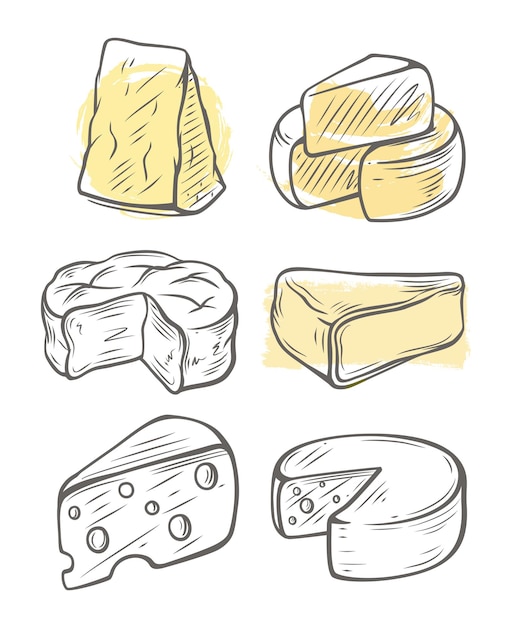This image is a set of six line drawings depicting various types of cheese, presented in a simple black on white background with selective shading in yellow. The drawings are arranged in three rows, each featuring two different cheeses that are either wedges or rounds. The top row includes a yellow-shaded wedge standing on its large side next to a yellow round with one slice cut out of it. The second row mirrors this arrangement: a round of cheese with a slice missing, both shaded in yellow, is on the left, with the yellow slice placed to the right. In the bottom row, there is a tall slice of Swiss cheese standing on its long end to the left, with an unshaded round of Swiss cheese with a slice removed situated to its right. The illustrations are done in a detailed sketch style with intricate line work in dark charcoal gray, complemented by subtle yellow accents to highlight certain pieces.